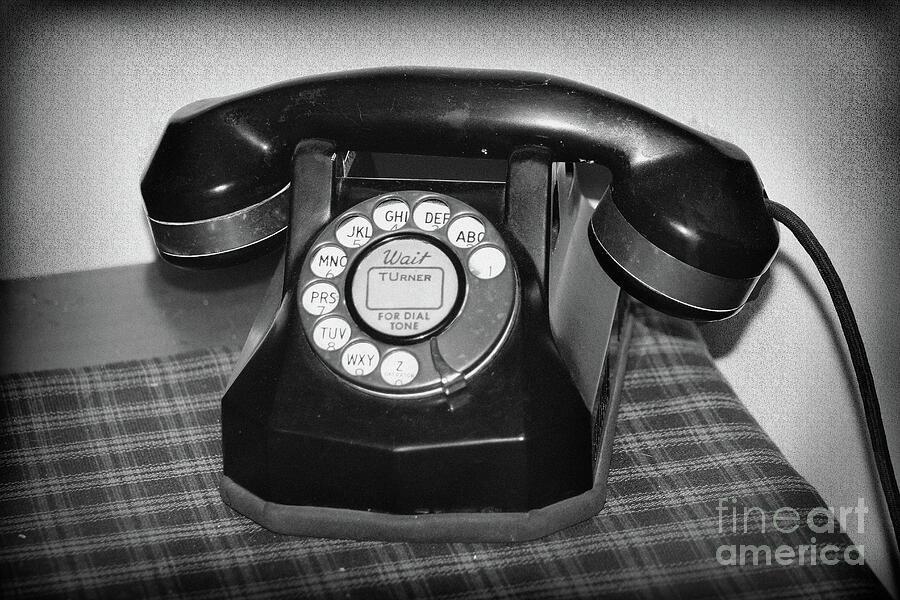This black-and-white photograph prominently features an old black rotary telephone, complete with a heavy handset and a thick cord connecting it to the base. The telephone, which has the letters of the alphabet around the numbers on the rotary dial, bears the text "Wait for dial tone" and "Turner." The phone rests on a wooden table covered with a striped or plaid fabric. The background is a grayish hue, enhancing the vintage aesthetic of the image. In the bottom right corner, the photograph is marked with the text "Fine Art America," adding a touch of authenticity and fine art appeal to the scene.